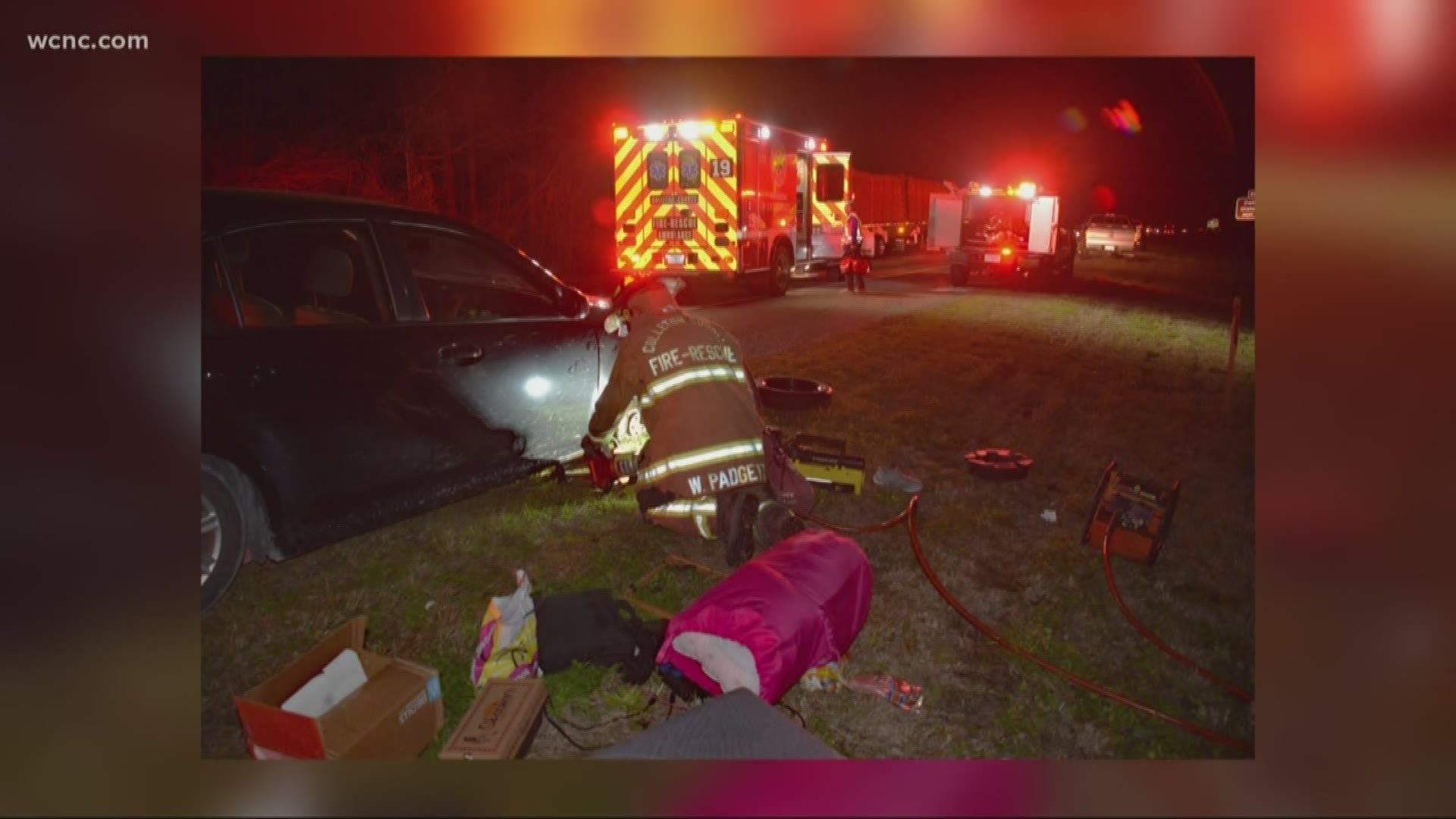The nighttime roadside emergency scene, captured from WCNC.com, depicts a firefighter, identifiable by the "fire rescue" label on his jacket, kneeling beside a black sedan that appears to have been in a crash. He is operating what seems to be the jaws of life, an orange hose trailing back to a generator. Scatterings of debris, including pink duffel bags, boxes, and other equipment, surround him. The image is well-illuminated by the flashing lights of an ambulance and possibly another emergency vehicle in the background. Additional emergency personnel and vehicles, like semi-trailers and trucks, are faintly visible, emphasizing the chaotic but controlled urgency of the scene.